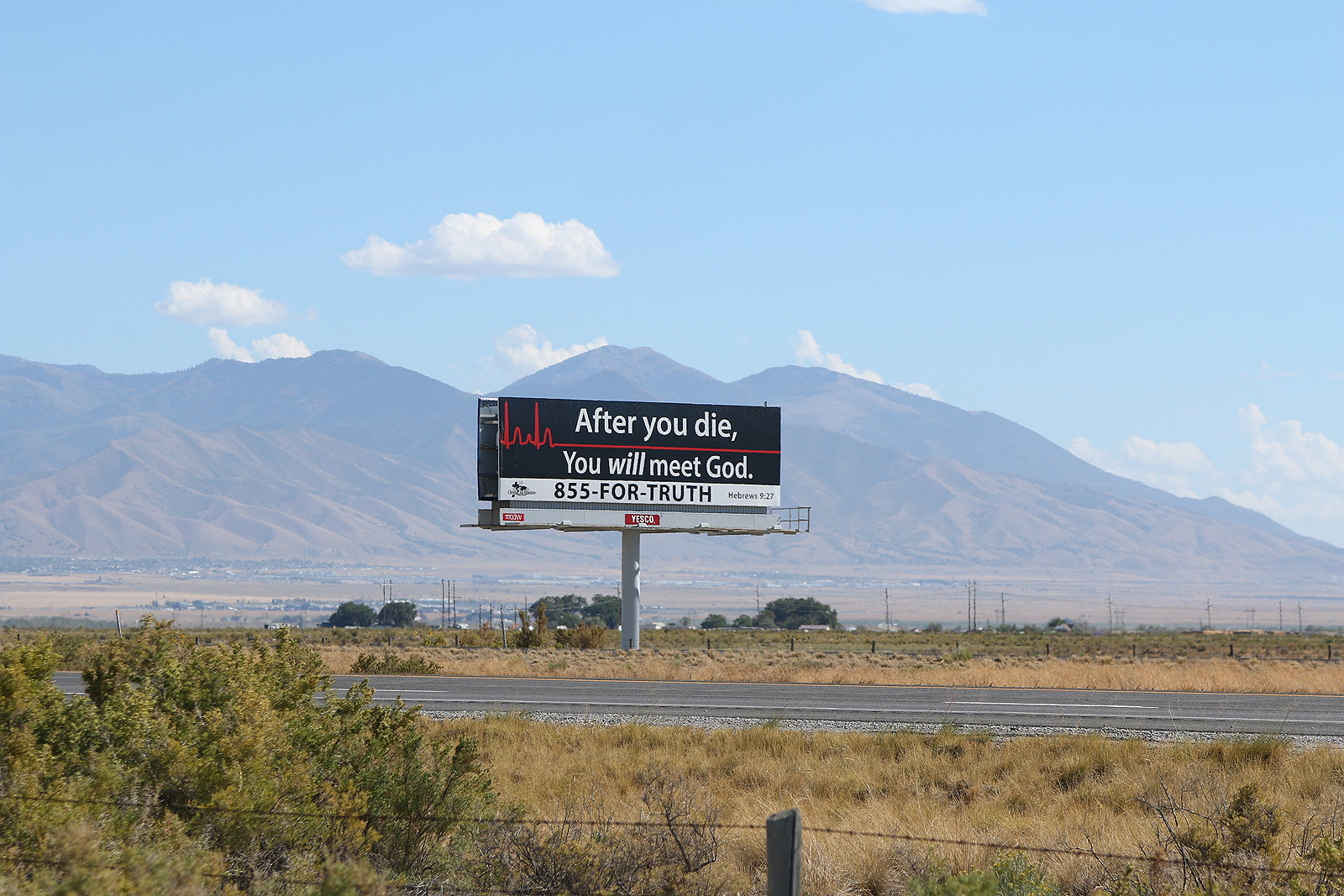The image features a prominently displayed billboard sign situated along a desolate roadside in a rural area. The billboard's background is predominantly black and features a graphic of a red heartbeat monitor line which transitions into a flatline, symbolizing the cessation of life. Centered on the billboard are the words, "After you die, you will meet God," followed by a call-to-action message and a phone number, "855-For-Truth." Below this, a Biblical reference, "Hebrews 9:27," is cited. The surrounding landscape is characterized by rolling hills, possibly large hills or small mountains, stretching into the background. The area appears very sparse and isolated, with no visible signs of vehicles or people on the road.